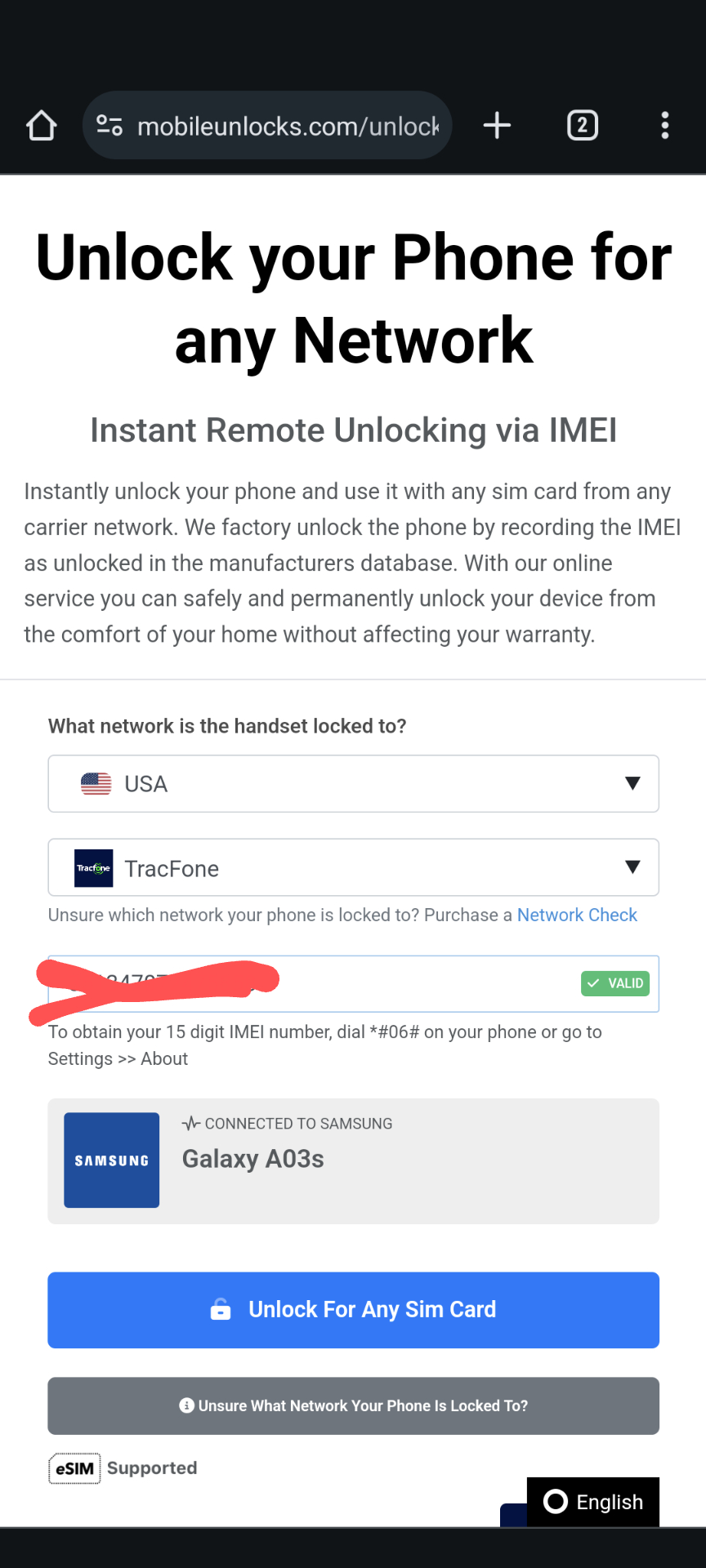**Detailed Caption:**

The image is a screenshot taken from a mobile phone displaying a webpage on the Google Chrome mobile app. The browser's user interface is visible with a black background. At the top left, the Chrome logo is displayed, and to the right, a plus sign allows adding new tabs, indicating the user is on the second tab, as shown by the number '2.' Further right, three vertically aligned dots present access to settings. 

The webpage in the screenshot is from "mobileunlocks.com/unlock," featuring a predominantly white background with black text. The headline "Unlock your phone for any network" stands out, followed by a description: "Instant remote unlocking via IMEI. Instantly unlock your phone and use it with any SIM card from any carrier network. We factory unlock the phone by recording the IMEI as unlocked in the manufacturer's database. With our online service, you can safely and permanently unlock your device from the comfort of your home without affecting your warranty."

Below the description, a prompt reads, "What network is the handset locked to?" accompanied by a USA flag logo with a dropdown menu. Another dropdown displays "TracFone" with an associated logo. There's an option highlighted in blue labeled "Purchase a network check," indicating it's a clickable hyperlink.

Partially obscured by red markings, a set of digits with a green background labeled "valid" appears. Instructions follow: "To obtain your 15-digit IMEI number, dial *#06# on your phone, or go to settings > about."

A Samsung advertisement is underneath, with the text "Connected to Samsung Galaxy A03s." Below, there are two rectangular buttons: a blue one labeled "Unlock for any SIM card" and a gray one for confirming the network your phone is locked to, labeled "Ensure which network your phone is locked to."

Further down, the text "eSIM supported" appears, and the bottom right corner of the screen shows the language selection as "English." Finally, a thick black bar spans the bottom of the screenshot.